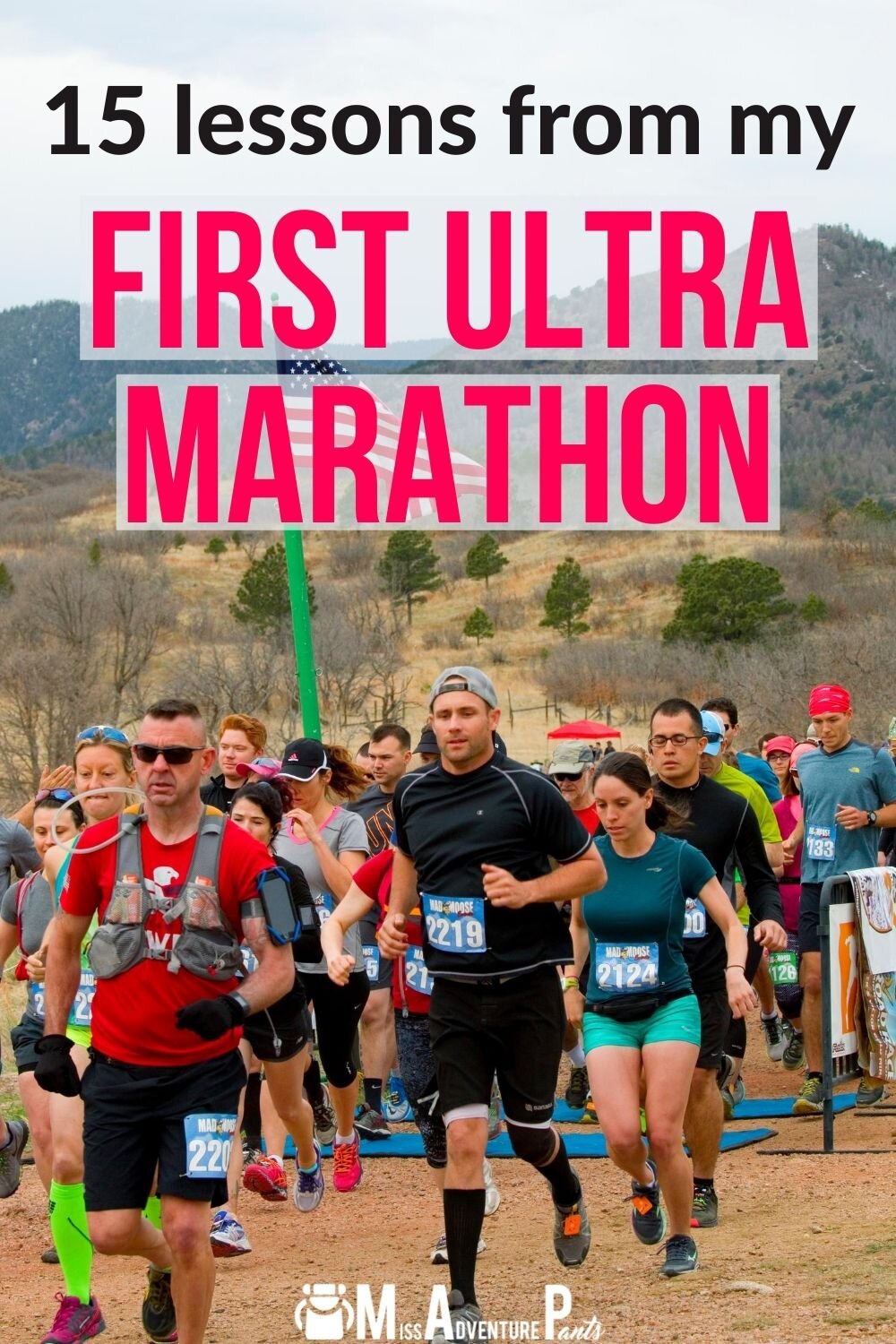This poster, reminiscent of something you might find on Pinterest, is designed to advertise an article titled "15 Lessons from My First Ultra Marathon." At the top, the title is presented in a combination of black font for "15 lessons from Mai" and striking pink font for "FIRST ULTRA MARATHON," both set against a light opaque white background. The central image captures a dynamic outdoor scene featuring a group of fit and determined runners, all adorned with race bibs displaying different numbers. The athletes are dressed in various workout clothing, including colors like black, teal, lime green, and red. Notable details include a woman in teal shorts paired with a black shirt, a man clad in red with black shorts, another runner sporting a backwards baseball cap, and some even accessorized with sunglasses and hats. The race appears to be taking place on a rugged outdoor trail, evident from the cross-country landscape and a runner proudly holding an American flag. Adding an adventurous spirit to the poster, the bottom of the image features white text that reads "Miss Adventure Pants," further emphasizing the theme of exploration and endurance.